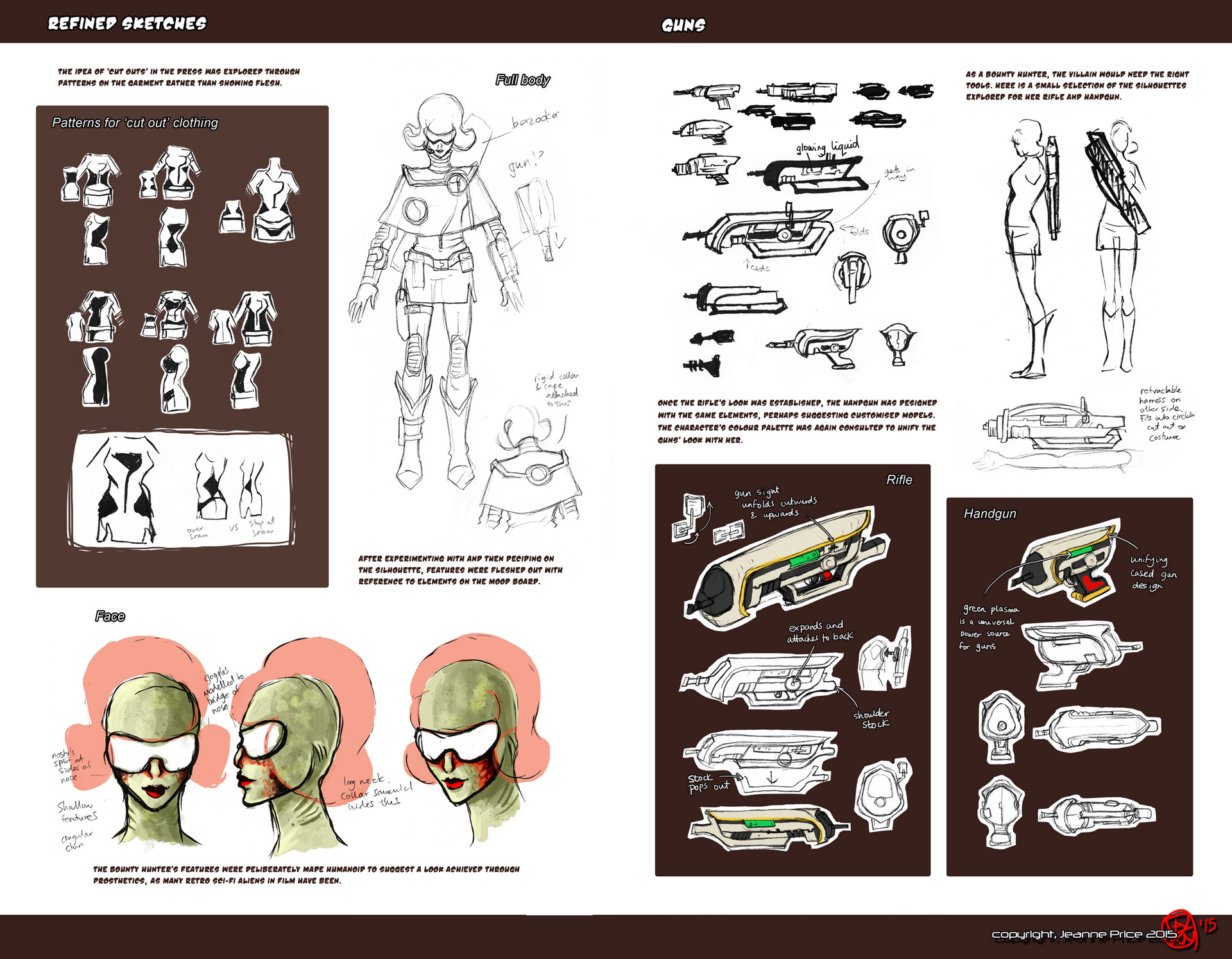The image is a detailed sketch diagram poster, prominently featuring a layout of various designs and diagrams against a white background. At the top left, within a brown banner, it bears the title "Refined Sketches" with the word "Kung" prominently displayed in the center. Below this banner, to the left, there's a large brown rectangle titled "Patterns for Cut Out Clothing," containing several diagrams. Adjacent to this is a full-body sketch, possibly of a person wearing a futuristic spacesuit. Below, in the bottom left corner, a series of three angles of a face mask are featured, labeled "Face" in small black letters. On the right side of the poster, there are detailed sketches of various weapons, including a section in the lower right that showcases rifles with accompanying diagrams inside a brown rectangular box labeled "Rifle" in the top right corner. Further down in the bottom right, another brown rectangle illustrates sketches of handguns. In the bottom right corner, yet another brown banner contains "Copyright" alongside a name and a logo, adding a formal touch to the intricate and highly detailed designs that span the entire poster.